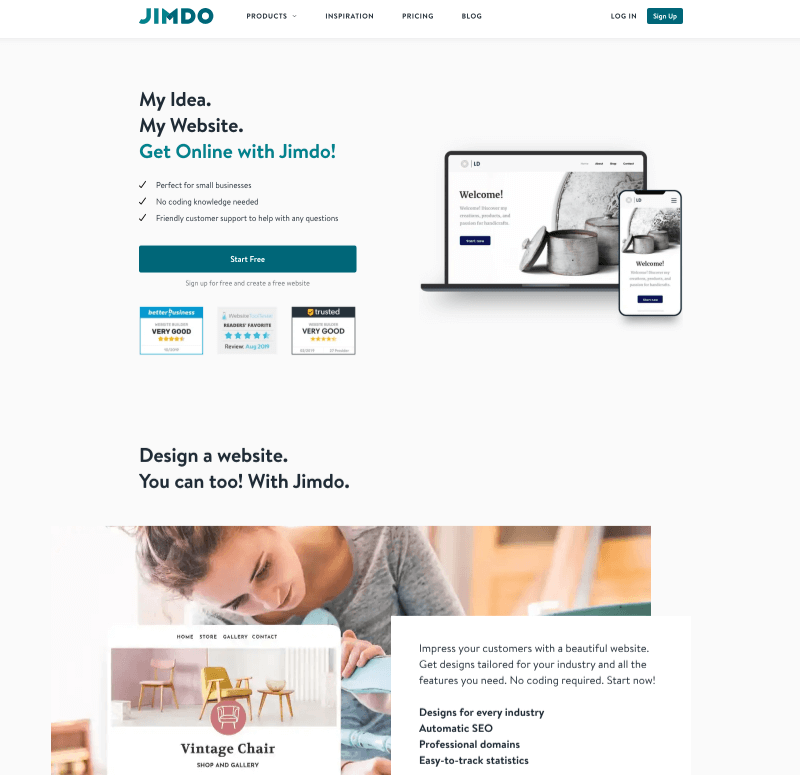A website landing page is displayed, highlighting GIMDO's product offerings. The top banner reads "Welcome to Tech," followed by various icons and a header with product links such as Inspiration, Pricing, Blog, Login, and Sign Up. Below, a smartphone image is prominently featured, alongside a blue rectangle button prompting "Start Free" and "Create a Free Website." Additionally, there's an annotation about the service being highly rated, with "Readers’ Favorite: 4.5 Stars out of 5," along with claims of trusted and good design.

To the right, there is a testimonial quote: “Design a website you can too with Jim Doe." Below this, a woman is seen looking down at something not fully visible. The site navigation bar includes options like Home, Story, Gallery, and Contact. An indoor scene shows two vintage chairs and a small table with a bowl on top, likely part of the "Gallery" section. A red circle highlights a section with more details about the vintage chairs. The right sidebar notes, "Impress your customers with a beautiful website designed for your industry, with all the features you need. No coding required. Start now!"

Additional features include bullet points for "Designed for every industry," "Automatic SEO," "Professional domains," and "Easy-to-track statistics." The overall aesthetic is user-friendly with prominent features aimed at small businesses and those without coding knowledge, underscoring GIMDO’s supportive customer service and comprehensive website-building tools.